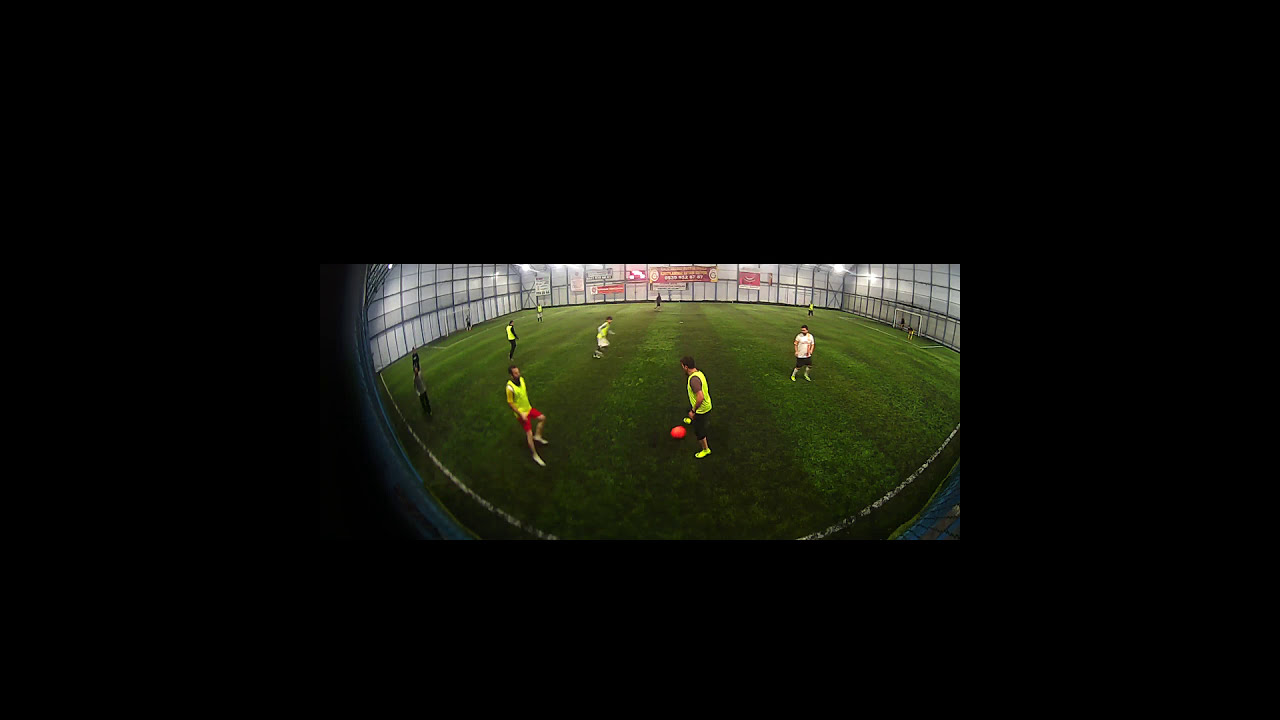The image depicts an indoor soccer facility with a distinctly warped view, suggesting it was taken with a fisheye lens. In the middle center of the image is an inset photo of a team of soccer players on an indoor green turf field, which features alternating light and dark green stripes. Prominently in the foreground on the left third, a man donned in red shorts and a neon yellow top stands out. In the right center, another man in a matching yellow fluorescent top, black shorts, and white shoes is poised near a bright red soccer ball. The arena is enclosed with white walls, interlaced with a grid of black metal framing forming squares. Hanging on the back wall are red banners with white text. The entire scene is bordered by a black frame, encapsulating the vibrant colors: black, gray, red, purple, lime green, light blue, and dark blue. Despite the visual vibrancy and activity, there is no discernible text within the primary image itself. The setting is clearly indoors, marked by the grid lines along the top perimeter, suggesting an organized and enclosed sports venue.